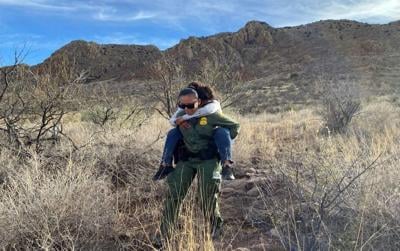In this color photograph, a woman is carrying a child on her back, set against a rugged, dramatic mountainous backdrop. The woman, dressed in a green long-sleeved shirt and pants with a black belt, has her brown hair pinned back and wears black sunglasses. The child's arms are tightly wrapped around her mother's neck, and though the child's face isn't visible, her attire includes blue denim jeans, black shoes, and a long-sleeved white shirt. They traverse a dirt path surrounded by sparse desert vegetation — predominantly brown, gray, and yellow colors dominate the scene, with brush, high grasses, and a leafless tree visible. The mountains in the background are large and rocky, casting a formidable presence below a sky that is light blue with scattered white clouds. The image is textless and lacks overt context, suggesting it could be either a spontaneous moment or an intentionally serene capture of day-to-day life.